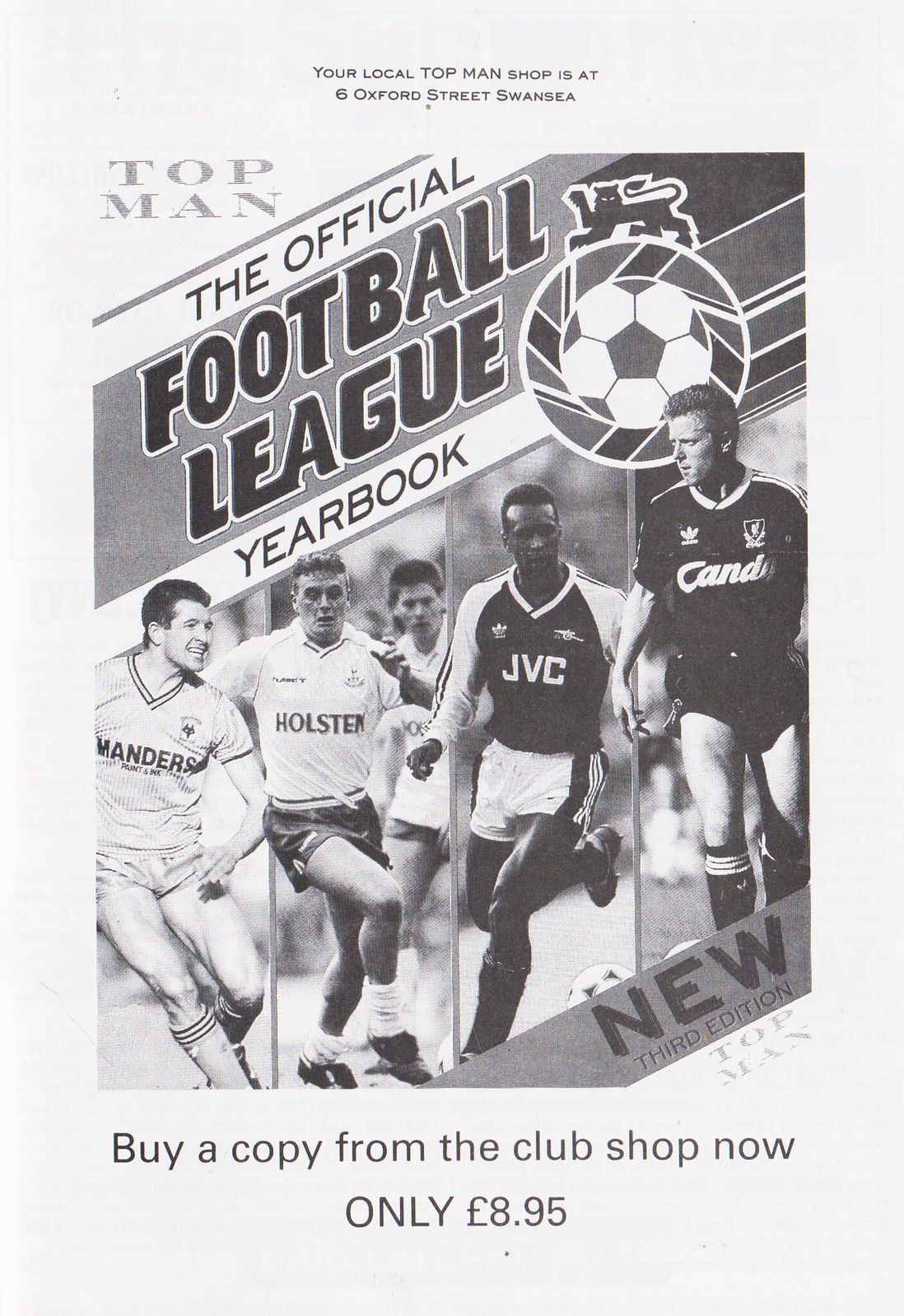The image is a black-and-white magazine cover for a soccer yearbook. It features a central photo of various soccer players arranged from left to right. The cover has multiple textual elements meticulously distributed across its white backdrop. At the top, small black text reads, "Your local Top Man shop is at 6 Oxford Street, Swansea." Below this, two upward-angled text bands proclaim "The Official" and "Football League," respectively, with "Football League" rendered in a striking black font outlined in white against a grey background. Further down, the word "Yearbook" stands in black against a white background, accompanied by a classic black-and-white soccer ball to its right. The bottom of the cover is accentuated by a grey band that runs across the bottom right corner, boldly declaring "New Third Edition" in black lettering. Below this band, additional text instructs, "Buy a copy from the club shop now, only £8.95." This cover serves both as a promotional advertisement and an informative display, emphasizing the new third edition of the official football yearbook brought to you by Top Man.